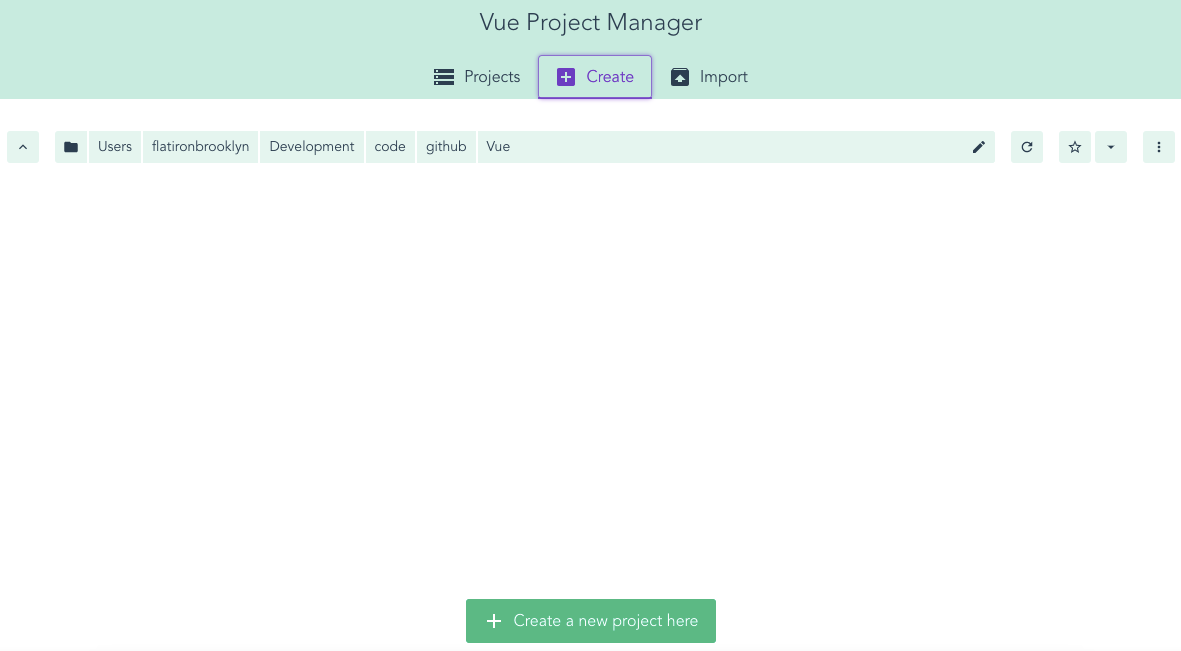The image displays a user interface for a project management tool. Across the top, a light bluish-green banner prominently features the text "View Project Manager" positioned at its center. Below the banner, three vertical lines separate different sections.

In the central area, there is a purple square divided by a cross, with the word "Create" inscribed within it. This square is bordered by a rectangle. Adjacent to this is another section labeled "Import," highlighted by an icon featuring a classic upward-pointing arrow within a black box.

Further down, the interface presents several options arranged in a list, including folders and labels for "Users," "Flatiron Brooklyn," "Development Code," "JitHub," and "View." There is also a pencil icon, presumably indicating an editing function.

The bottom portion of the interface is predominantly white, suggesting no projects have been created yet. At the very bottom, a green rectangular button with a white cross in its center invites the user to "Create a new project here." The overall impression is that this is a blank workspace awaiting the user's input to create or import projects.